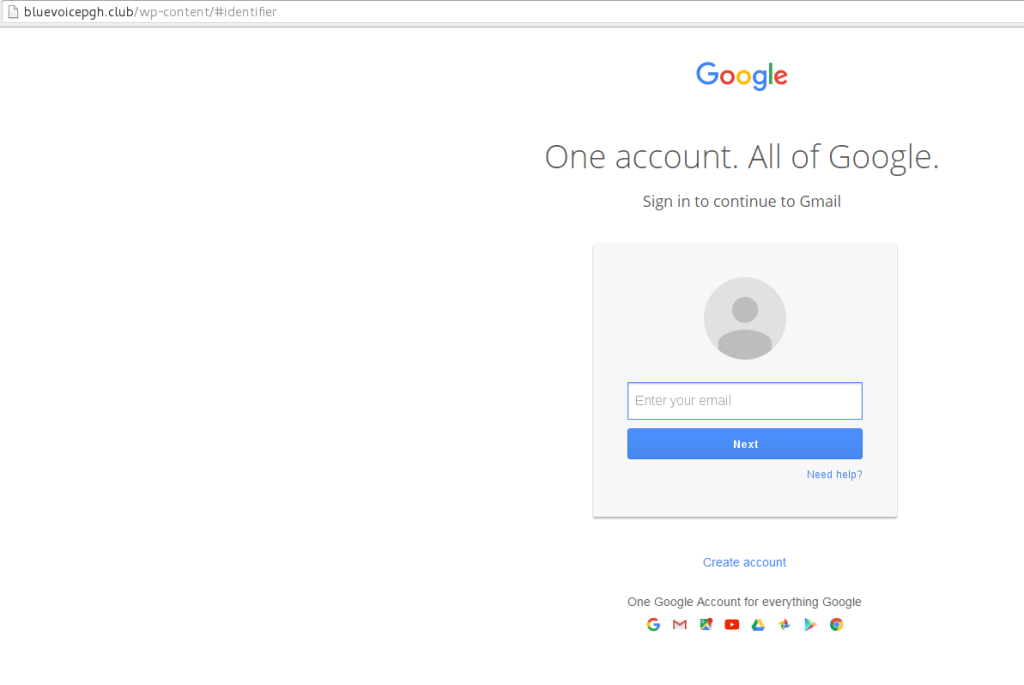The screenshot depicts a laptop screen displaying a web browser with the URL indicative of a website potentially related to "Blue Voice PGH," likely an abbreviation for Blue Voice Pittsburgh. The URL path includes “wp-content,” suggesting it is a WordPress-based site. Despite the URL, the main content visible on the screen is a Google sign-in page.

The Google page prominently features the familiar rainbow-colored Google logo, accompanied by the text, "One account. All of Google." Below this phrase is an instruction to "Sign in to continue to Gmail." A floating dialog box brands an icon of a person and contains a text field labeled “Enter your email” with a button labeled “Next.” Additional options include a "Need help?" link and a "Create account" notice, which is outside but associated with the dialog box. The page reassures users with the message, "Just one Google account for everything Google."

The presence of the Google sign-in page causes some confusion given the URL suggests the user is visiting the Blue Voice Pittsburgh website. This juxtaposition suggests a possible misdirection or an unexpected redirection, leading to ambiguity about the exact nature of the site being accessed.